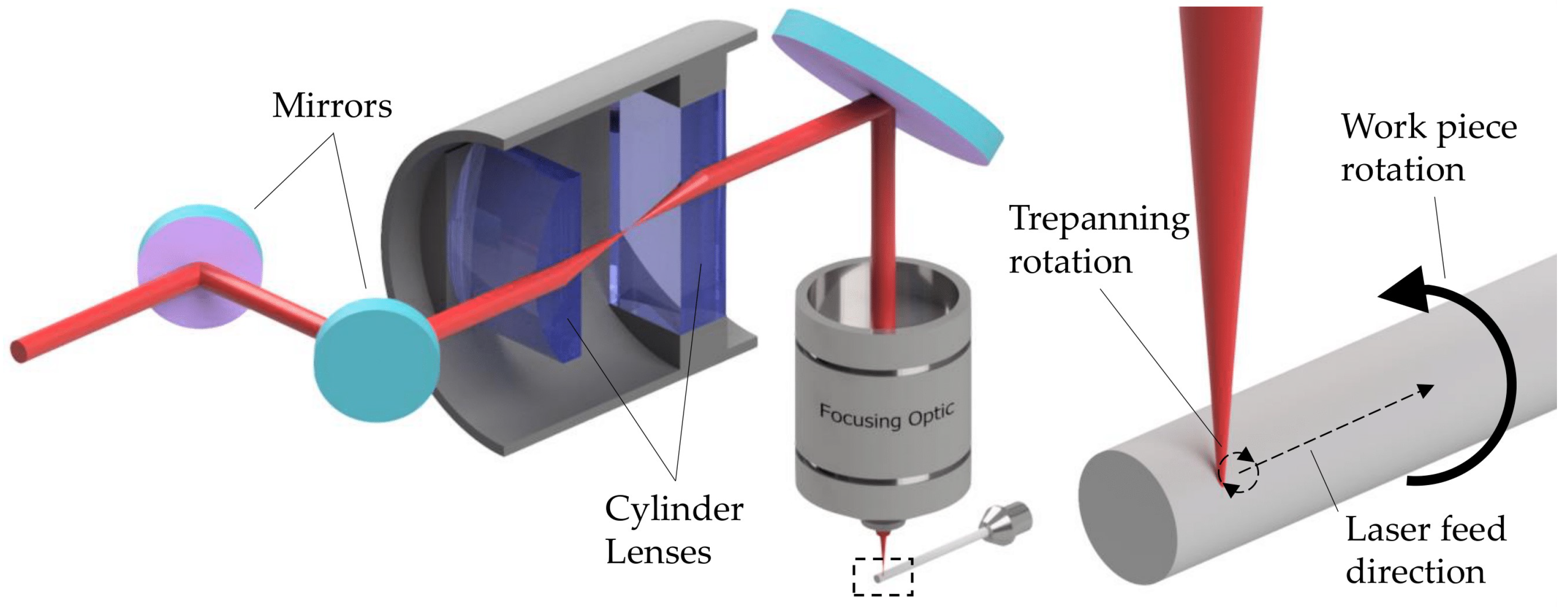The diagram depicts a detailed schematic of a cylindrical apparatus engaged in a laser etching process. On the left side of the image, the interior of the primary cylinder is visible, revealing two blue, glass-like objects labeled as cylinder lenses. Externally, two round objects identified as mirrors interact with a red laser beam, which reflects off the mirrors before passing through the lenses. The laser beam subsequently strikes another mirror, directing the beam into a secondary cylinder labeled as a focusing optic, which appears to have a metallic interior.

The diagram transitions to a close-up view of a metal rod situated beneath the focusing optic, where the laser beam is actively etching a circular pattern onto the rotating rod. The technical annotations include terms such as 'tree-panning rotation,' 'workpiece rotation,' and 'laser feed direction,' illustrating the laser's path and interaction with the rod. These components suggest a sophisticated mechanism, potentially for precise laser machining or etching, though the exact application remains unclear from the provided context.